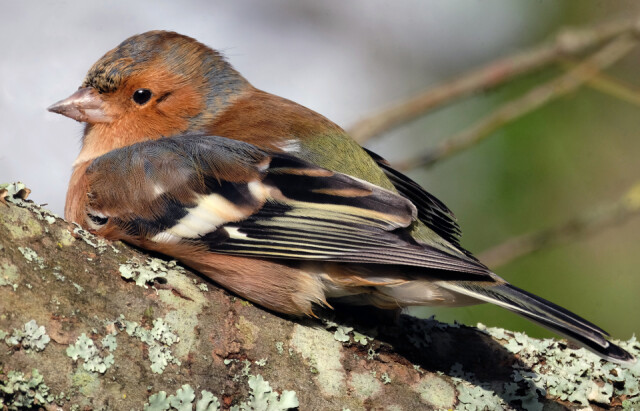This detailed photograph captures a small bird, likely a sparrow, perched on a lichen-covered brown tree limb. The bird features a short, slightly pointy beak and a striking orange face, with its black eye visible in profile. Its plumage showcases an assortment of brown and green on its back, while its wings are a mix of gray, brown, and white, and its extended tail appears to be black. The bird's fine feathers give it a texture almost like fur, contributing to its somewhat fluffy, palm-sized appearance. It gazes slightly to the lower left, bringing a hint of curiosity to its demeanor. The background, softly blurred, reveals vague shapes of additional tree branches, green foliage, and possibly some sky, emphasizing the focus on the bird itself.